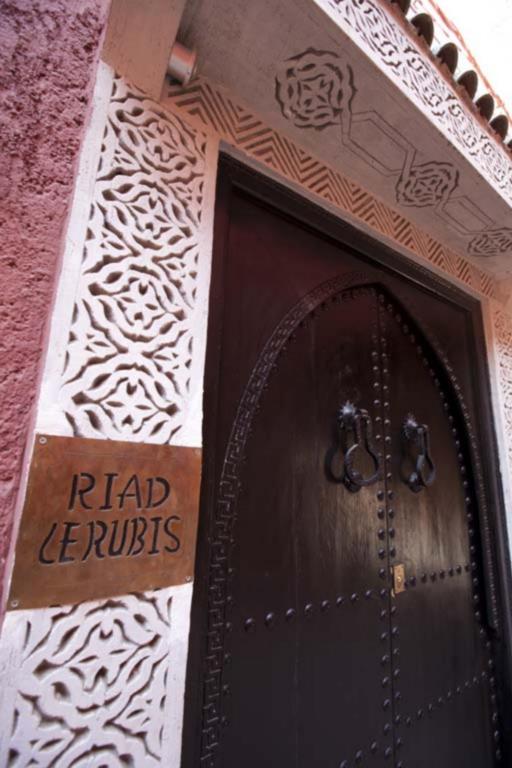This image showcases the ornate entryway of a prestigious and elegant building, possibly a Riad named "Riad Lerubis". The entrance is framed by a highly detailed stone archway, intricately carved and decorative, which enhances the grandeur of the scene. This archway has a stone or ceramic ledge above it, adorned with elegant, possibly rose-like designs, contributing to its elaborate appearance.

The focal point of the image is a pair of massive, dark brown metal doors almost black in color. These doors are extensively decorated with intricate embossing and carvings, featuring a riveted pattern forming oval shapes reminiscent of window panes. Large, imposing door knockers are prominently attached, highlighting the doors' robust craftsmanship. 

Adjacent to these magnificent doors, the exterior wall of the building is visible, displaying a natural pinkish-red clay hue that complements the rich tones of the entryway. A copper or brass sign is mounted nearby, bearing the name "Riad Lerubis" in black lettering, indicating the identity of this esteemed structure.